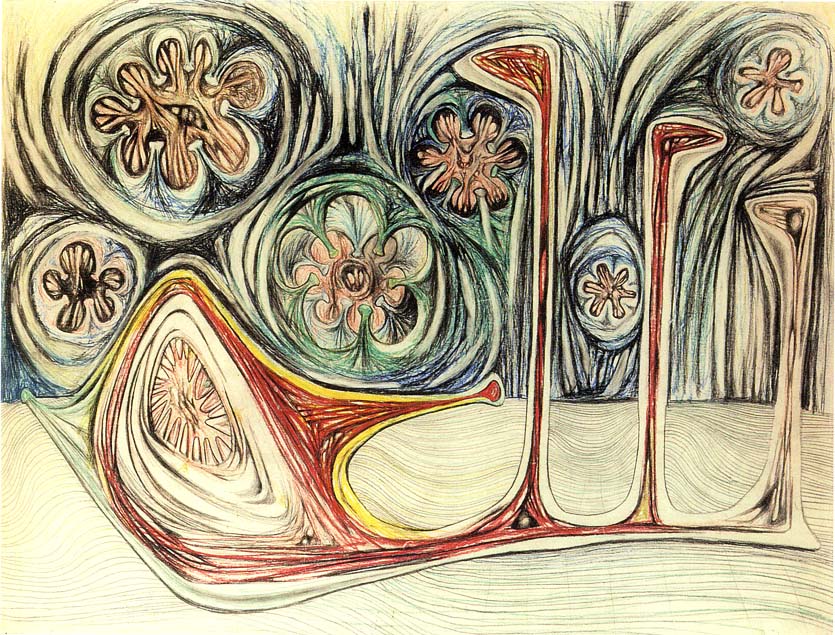This abstract modern print features a vivid and intricate interplay of shapes and colors. Dominating the bottom of the image is a prominent red form, reminiscent of a mouth with teeth, tapering into a triangular shape that culminates on the left side of the picture. In the center of this triangle sits a striking circular feature. Surrounding this central shape are numerous spherical figures of varying sizes and colors, including red, yellow, green, blue, and white. These spheres contain interior designs that resemble smaller interconnected spheres, connected aesthetically like spokes on a wheel.

Intricately weaving through the image are a plethora of lines and curves, forming flower-like patterns. Inside some of these flowers, small details resemble eyeballs, mouths, or faces, though this perception could vary, suggesting an organic, almost alive quality to the entire composition. This movement is echoed by vertical, lamp post-like shapes that stretch upward from the triangle's base towards the background.

Overall, the image is rich in layers and textures, inviting a multitude of interpretations—from vibrant, abstract florals to cellular structures or whimsical, puzzle-like formations. This captivating print is a harmonious blend of color, form, and motion, leaving its full meaning open to the observer's imagination.